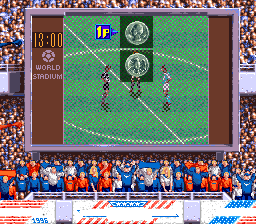The image displays a detailed scoreboard from a video game. Surrounding the scoreboard are animated fans dressed predominantly in blue and red attire, giving a lively atmosphere to the scene. The fans appear to be Caucasian in complexion. At the bottom of the screen, the year 1996 is prominently displayed in blue font.

The background features a white wall adorned with alternating red and blue stripes. In the center of the screen, on the left side, there are brown edges framing the display. The scoreboard itself includes the words "World Stadium" in white text alongside the Plymouth logo.

Highlighted in orange text is a timer showing 13 minutes. The main area of the screen replicates the markings of a soccer field, featuring a large white circle bisected by a straight line, symbolizing the center of the field. Depicted in the center are two players positioned on opposite sides of a coin, indicating a coin toss scenario. A blue square, marked with "1P" in yellow, points to the heads side of the coin. The right side of the screen mirrors the left with matching brown borders framing the scoreboard.